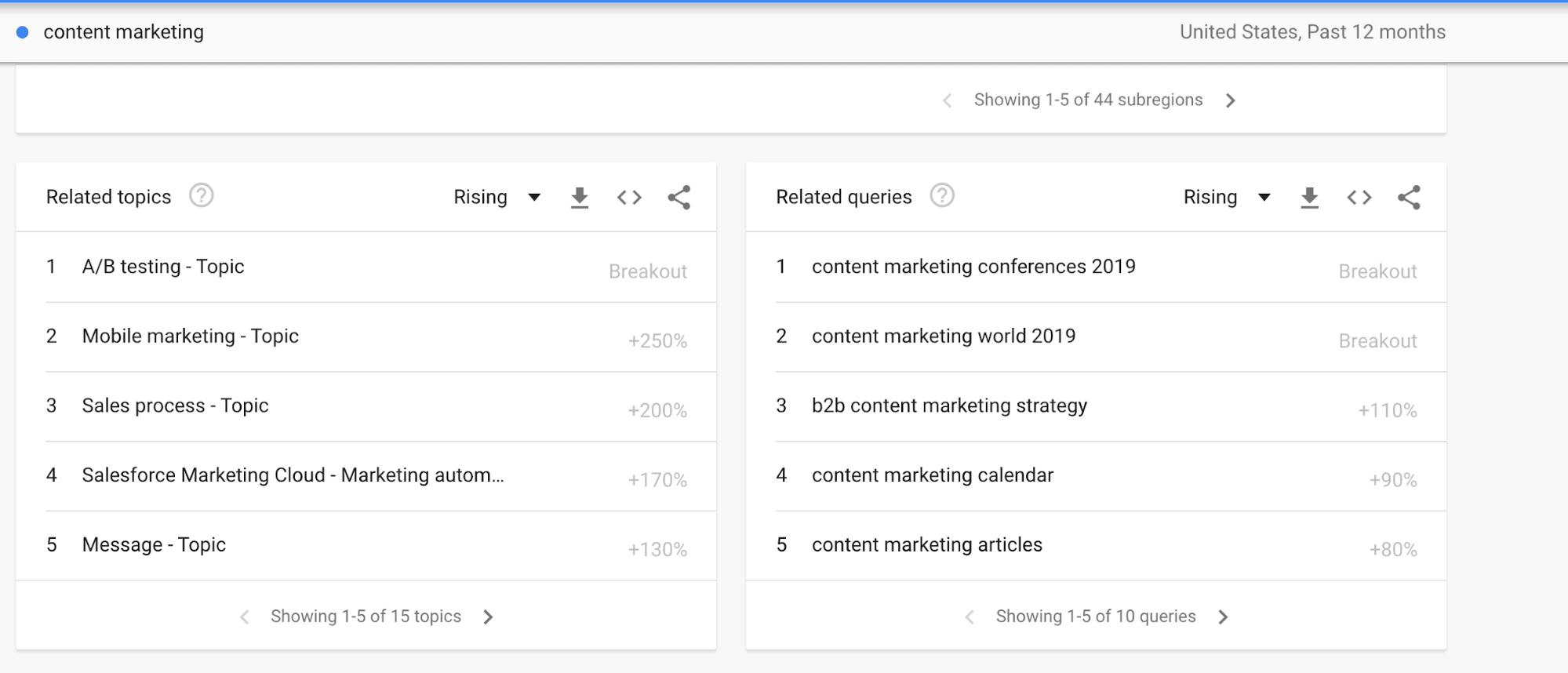This image illustrates a detailed dashboard for analyzing content marketing trends in the United States over the past 12 months. 

At the top, a prominent dark blue line serves as the header. Just below this header, a large blue circle prominently features the text "Content Marketing." To its right, the phrase "United States, Past 12 Months" is clearly displayed. 

Below this section, a light gray line spans the width of the dashboard, providing a subtle division. Directly underneath, there's a white box. Inside the white box, on the right side, the image indicates that it shows "1 of 5 / 44 subregions." 

Further down, there is a light gray area containing two white boxes positioned side by side. The left box is titled "Related Topics." Under this title, it lists several topics:
1. A/B Testing
2. Mobile Marketing
3. Sales Process
4. Salesforce Marketing Cloud - Marketing Automation
5. Messaging Topic

To the right of the "Related Topics" box, the white box is labeled "Related Queries." Listed below this label are:
1. Content Marketing Conferences 2019
2. Content Marketing World 2019
3. B2B Content Marketing Strategy

The image clearly demonstrates a comprehensive breakdown of related topics and queries associated with content marketing, presented in a well-structured and visually organized manner.